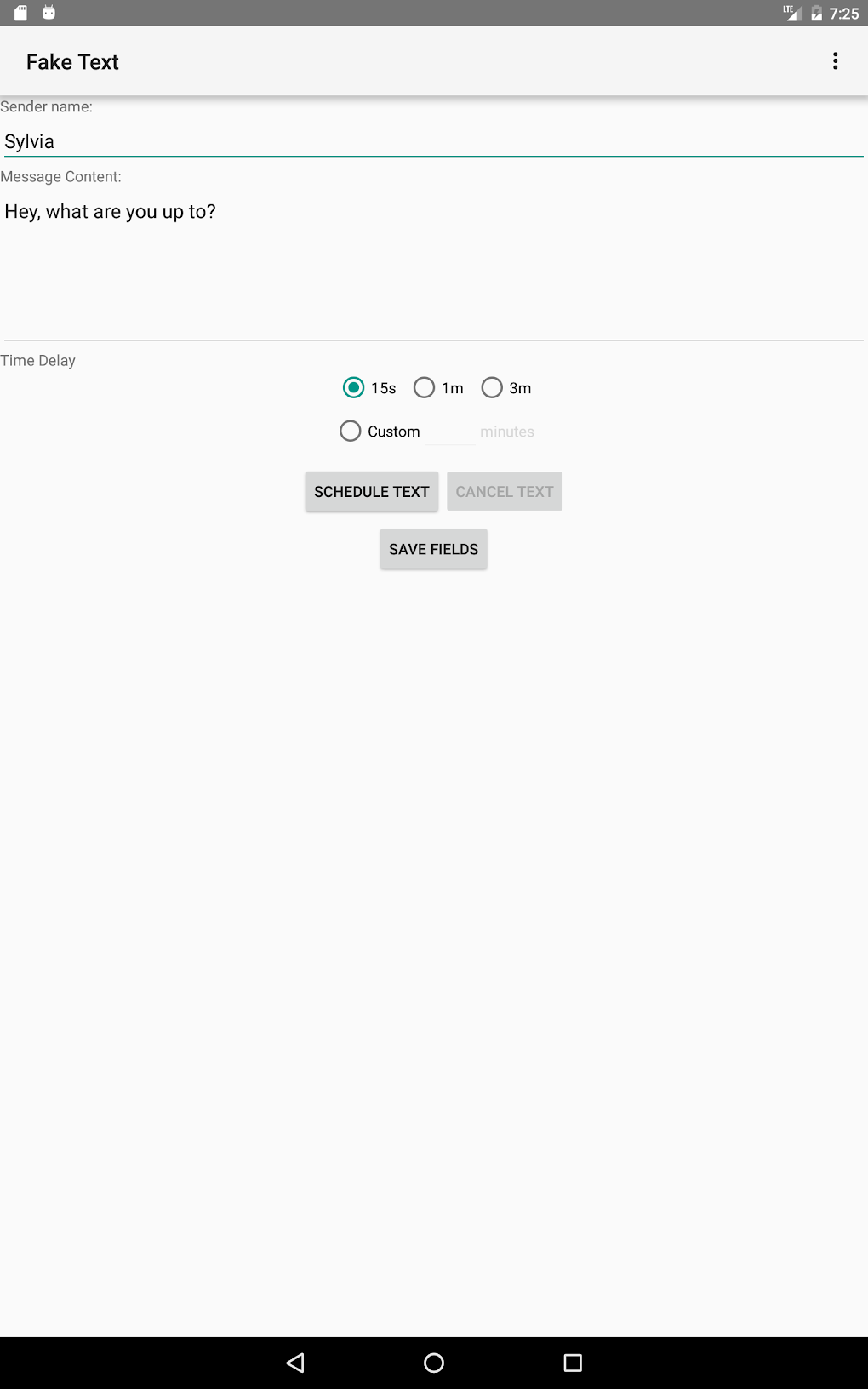The image depicts a computer screen interface designed for sending a scheduled text message.

At the top of the screen, bold text reads "Fake Test." Beneath this heading, another label says "Sender Name," with the name "Sylvia" entered in the adjacent field. A bluish-green horizontal line spans the width of the screen, visually separating sections.

Below the line, there's a label for "Message Content," and the text input area contains the message: "Hey, what are you up to?" in black font. An expansive blank area follows this text box, leading to a faint gray horizontal line that stretches across the screen.

Below this line, the label "Time Delay" appears, next to a circular button marked "15s" indicating a 15-second delay. Additional options labeled "1m" (1 minute) and "3m" (3 minutes) are clickable buttons positioned alongside. There is also a "Custom" option with a blank input field intended for users to specify a different time delay in minutes.

Further down, three gray rectangles with text are laid out, two at the top and one centered below them. The first rectangle is labeled "Schedule Text," the second "Cancel Text," and the third "Save Fields." The "Cancel Text" button, unlike the others, features gray text on a gray background, making it less prominent. The other two buttons display black text on a gray background.